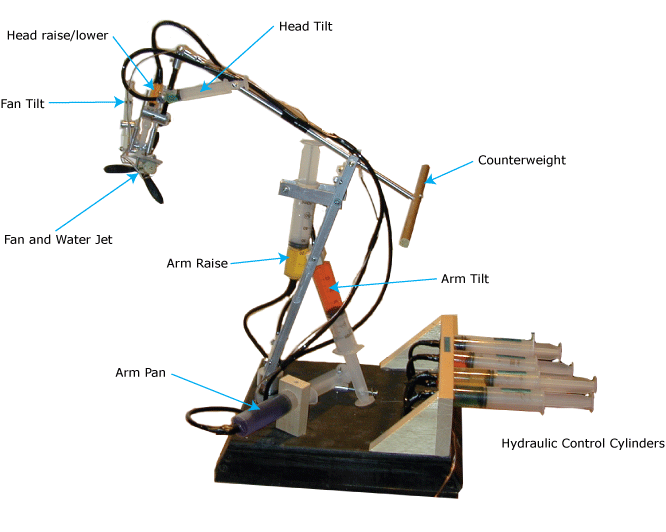In this detailed image of a science project, the contraption appears to be a model demonstrating the mechanics of hydraulics or a simple robotic arm. The project is set on a black square platform and features a variety of labeled parts connected to a series of colorful syringes, which serve as hydraulic pumps. The background of the image is white, providing a clear contrast to the device.

Starting from the bottom right corner and moving clockwise, the labels identify the components as follows: hydraulic control cylinders, arm pan, arm raise, fan and water jet, fan tilt, head raise/lower, head tilt, counterweight, and arm tilt. The robotic arm on the left side of the platform, which includes multiple joints and elbows, ends with a fan and water jet. Blue arrows on the contraption guide the viewer through these labeled parts, enhancing understanding of each component’s function.